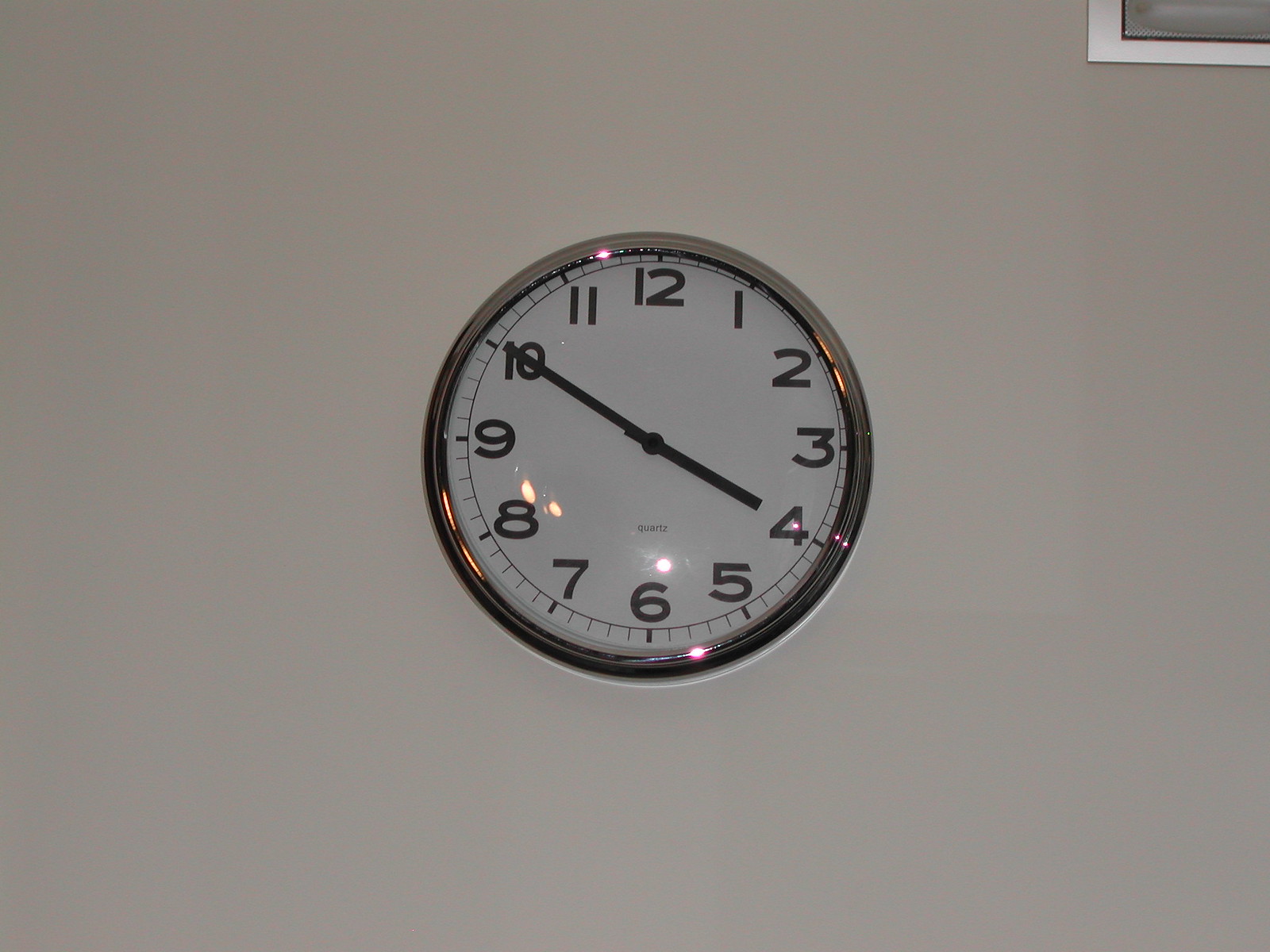The image depicts a slightly underexposed color photograph of a light grayish-beige-pastel toned wall. At the very center of the image, a round wall clock dominates the scene with its reflective silver frame, chrome-like in its ability to capture and highlight light, featuring subtle pink and orange reflections. The clock face is white, with black hands set to 3:50, large black numerals, and minute markers. The words "quartz" in small black text sit beneath the hands' central axis. The wall is otherwise unadorned, lending an emphasis to the clock. In the top right corner of the image, there is a small, rectangular feature on the wall, possibly a window or similar structure, faintly noticeable with a white border. The clock face displays notable glare with approximately five highlighted reflections from lights, adding to the reflective quality of the image.